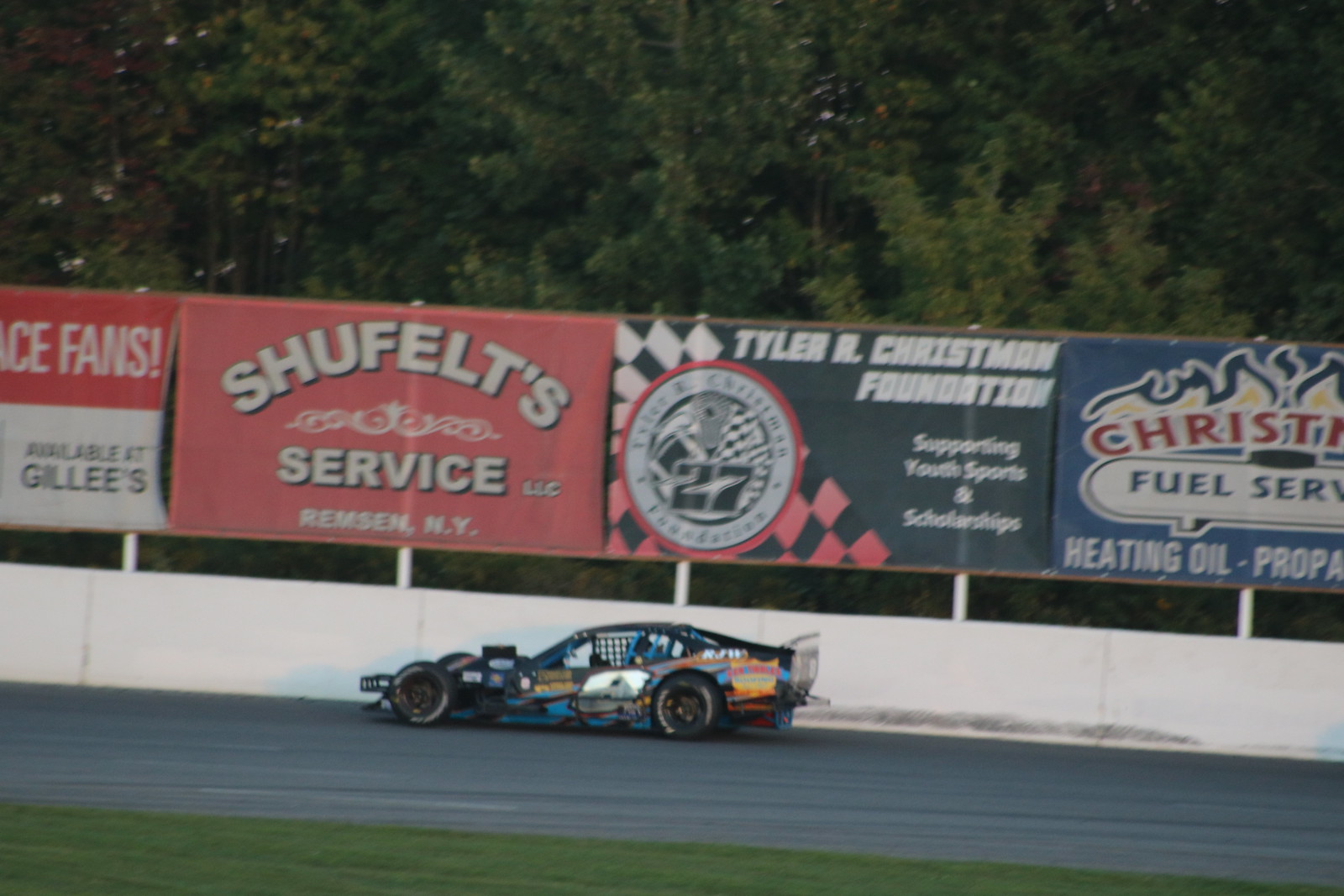The image depicts a dynamic scene of a black stock car with numerous decals, prominently featuring a gold number eight on its door, navigating a winding asphalt track. The action unfolds during the daytime, surrounded by a lush green field and an array of trees that enclose the track, creating a verdant backdrop. A stark white barricade lines the track, which, at one point, appears marked with black scuff marks, suggesting recent contact with the car.

Above the barricade are several advertising billboards and signs. On the left, a sign reads "Shoe Felt Service Remsen, NY." In the center, another billboard displays "Tyler R. Chrisman Foundation Supporting Youth Sports and Scholarships." A partially visible blue sign on the far right marks the end of this colorful display of sponsorships and ads. The overall scene vividly captures the thrill and environment of stock car racing, set against the serene yet vibrant surroundings of trees and a green field.